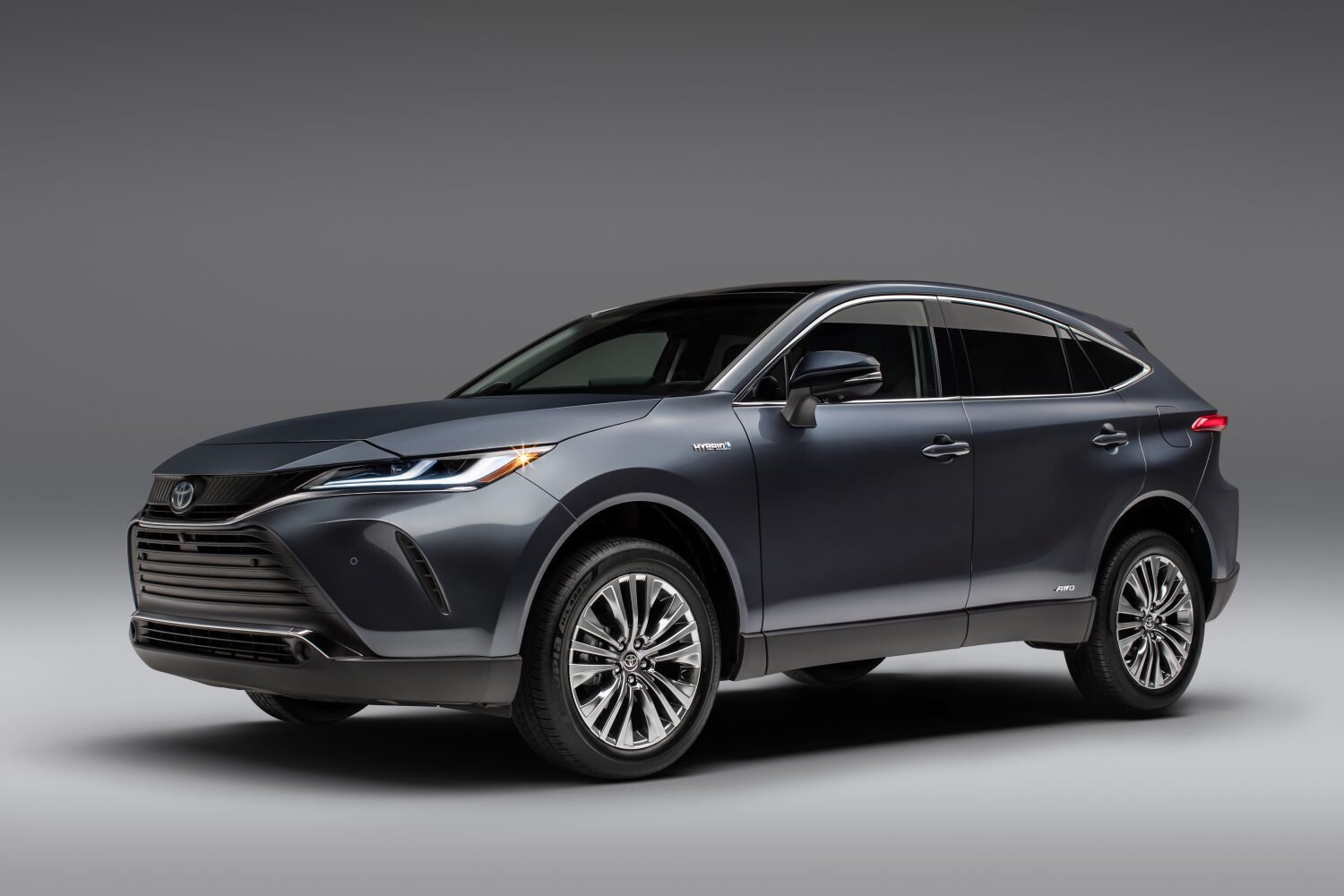The image showcases a sleek, modern SUV, primarily gray in color with vibrant accents of red, orange (possibly yellow), and black. The vehicle is positioned slightly turned towards the camera, which is angled from the front left. This mid-angle perspective allows a clear view of the Toyota emblem positioned between the headlights, indicating the brand. The SUV, marked as a hybrid with AWD (All-Wheel Drive) capabilities, features silver rims and lacks any visible license plates, suggesting it's a brand-new model potentially from 2024. The background is a clean, uniform gray, matching the floor and casting a shadow underneath the vehicle. No people are present in this high-quality advertisement photo, which is likely intended to highlight the vehicle's design and features for promotional purposes.